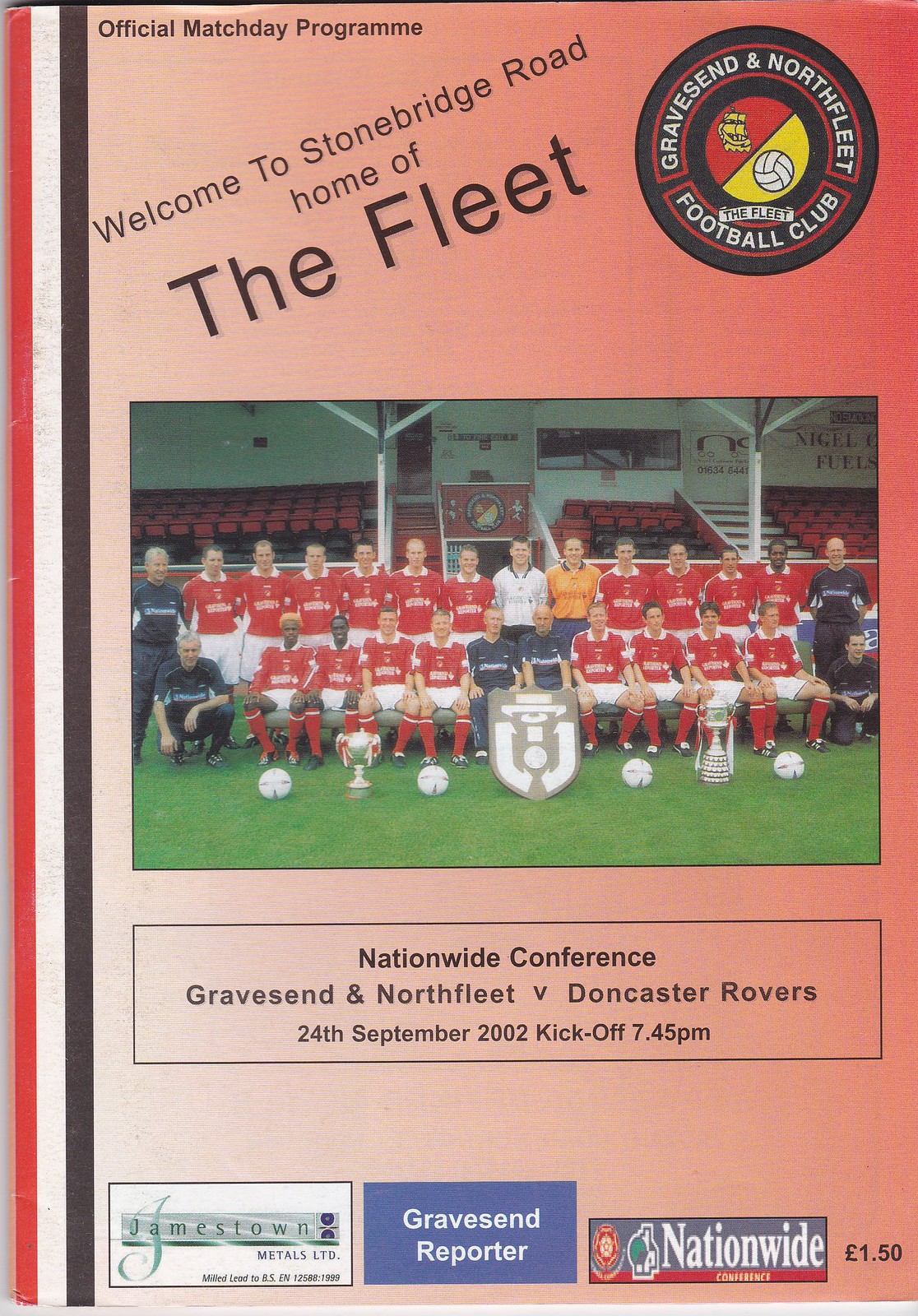The image depicts an official match day program for the Gravesend & Northfleet Football Club, referred to as "The Fleet," set against a pinkish-red background. The left side features a vertical border of red, white, and black stripes. At the top center, it reads "Official Match Day Program," followed by an angled text, "Welcome to Stonebridge Road, Home of The Fleet." On the upper right, there's a prominent black circle containing the club's name, "Gravesend & Northfleet Football Club," along with a soccer ball and a ship emblem. Centered below this is a team photograph showing two rows of players dressed in red and white, accompanied by coaches, with several soccer balls and trophies positioned on the grass in front of them. Beneath the photo, a black rectangle highlights the "Nationwide Conference" and details the match between Gravesend & Northfleet and Doncaster Rovers on September 24th, 2002, with a kickoff at 7:45 p.m. The bottom of the program includes ads for Jamestown Metals Limited, Gravesend Reporter, and Nationwide, and in the bottom right corner, the price is listed as 1.50 pence.